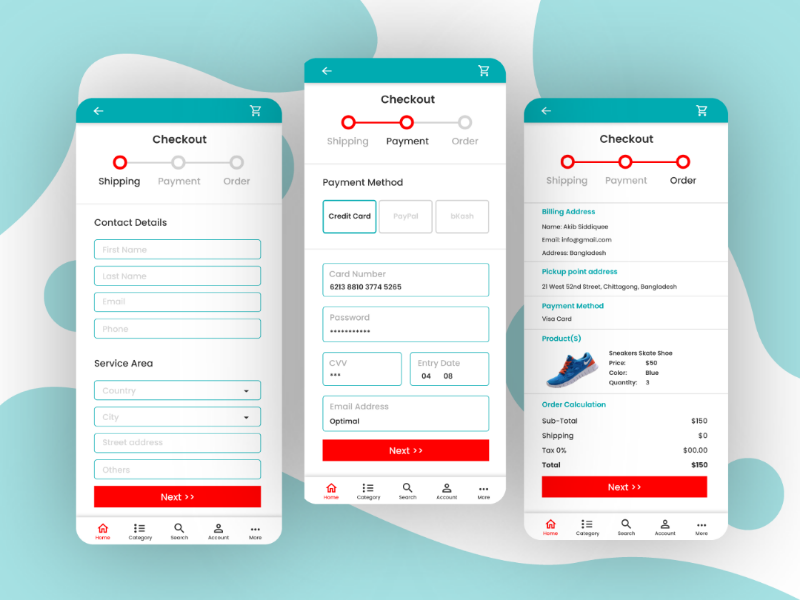This image provides a detailed view of the checkout functions for an online store. The process begins with the "Checkout - Shipping" section, where users are prompted to enter their contact details, including first and last name, email address, phone number, and service area, which requires county, city, and street address information.

Following this, the next section is dedicated to payment methods. Options include credit card and PayPal, though the image does not display all available methods. For credit card payments, users must input the card number, CVV number, expiration date, and optionally, an email address for receipt confirmation.

Subsequently, the order review section displays the billing address, pickup address, chosen payment method, list of products in the order, and a detailed breakdown of costs. This includes the subtotal, shipping charge, tax, and the final total amount.

The final step is to place the order, completing the checkout process. The image does not specify the website but indicates that the user is purchasing shoes, priced between $150 and $180.